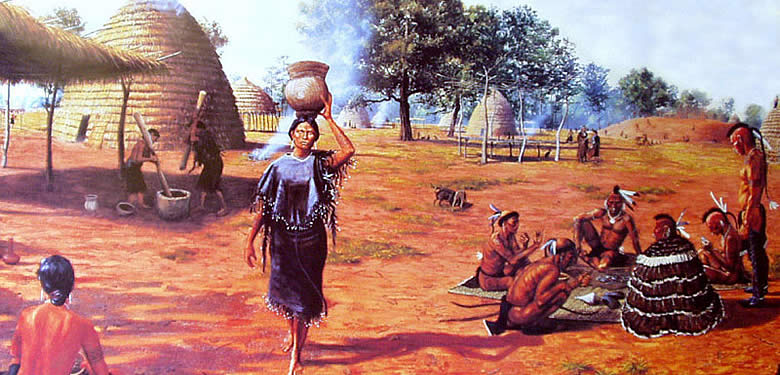The image is a vivid color illustration, possibly a painting, that showcases a Native American community in a southwestern setting. The ground is an orangish dirt, adding to the rustic ambiance. On the right side of the painting, a Native American woman, adorned in a dress with a cape top and a beaded skirt, walks toward the viewer. She gracefully balances a brown ceramic urn on her head with her left hand. To the lower right, six men, some wearing feather headbands and loincloths, gather in a circle on a blanket. Five are seated while one stands over them, and they engage in a communal activity. In the background, to the left, stands a dome-shaped hut made of grass and a teepee, with additional individuals actively churning something in a bowl with large sticks. This detailed scene captures the early lifestyles and habitats of the Caddo Indians in Tyler, Texas.